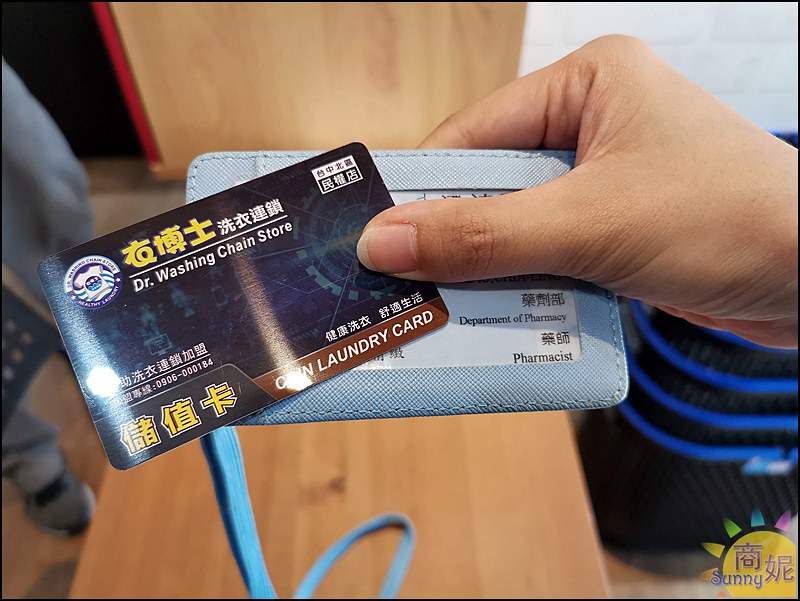In the image, a woman’s right hand holds a dark blue plastic card over a translucent blue wallet attached to a lanyard. The card bears Oriental characters in several places: at the top line, the bottom left, and the bottom right, as well as yellow Oriental characters at the very bottom. The text includes "Dr. Washington Store" and "coin laundry card," indicating it is likely used for laundry services in an apartment block. Behind the hand, a wooden table and a sliding wooden door against a white brick wall are visible in the background. To the left, there’s a plastic chair and legs wearing sweatpants and grey shoes, suggesting someone is standing nearby. The clear wallet itself reveals the words "Department of Pharmacy pharmacist" partially obscured below the thumb of the hand holding the card.